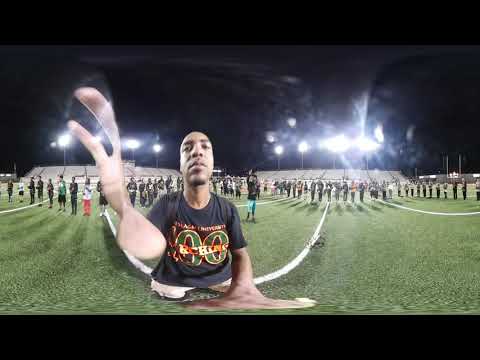The image is a horizontally rectangular photograph bordered by thick black lines at the top and bottom, taken with an unusual lens that significantly distorts the subject in the foreground. The scene is outdoors at night, on what appears to be a sports field with a grassy surface marked by white lines, possibly curbs or boundary markers.

Dominating the foreground is an African-American man, likely a performer or musician, wearing a black t-shirt displaying a "100" logo. His body and limbs are wildly distorted; his torso appears normal, but his raised left and right arms taper unnaturally, culminating in disproportionately large hands with elongated fingers. The foreground subject's position is slightly off-center, drawing immediate attention due to his unusual appearance.

Behind him, the background reveals a more defined setting of a nighttime event, possibly a parade or a school band performance. The green field is dotted with numerous people gathered around, though none are as close to the camera as the foreground subject. Flanking the field, bleachers are visible on either side, filled with spectators. Overhead, lights illuminate the scene, casting a bright glow on the crowd and highlighting the various colors present—black, green, tan, red, orange, yellow, white, and pink. The upper part of the image shows the night sky, completing the outdoor setting of this striking and surreal photograph.